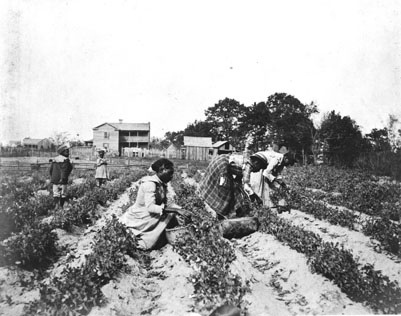The black and white photograph, which appears to be very old and not particularly clear, depicts a scene of laborers working in a field. In the background, there is an old farmhouse flanked by tall deciduous trees, with possibly barns and more houses visible. The sky above is a stark white. The field in the foreground is organized into roughly eight rows of crops with dirt pathways in between. Scattered throughout the rows are people, predominantly women and possibly some young children, who are kneeling or bent over, harvesting crops and placing them into baskets. This agrarian scene, marked by the long dresses worn by the workers and the presence of accompanying children, evokes a slice of rural life from a bygone era.